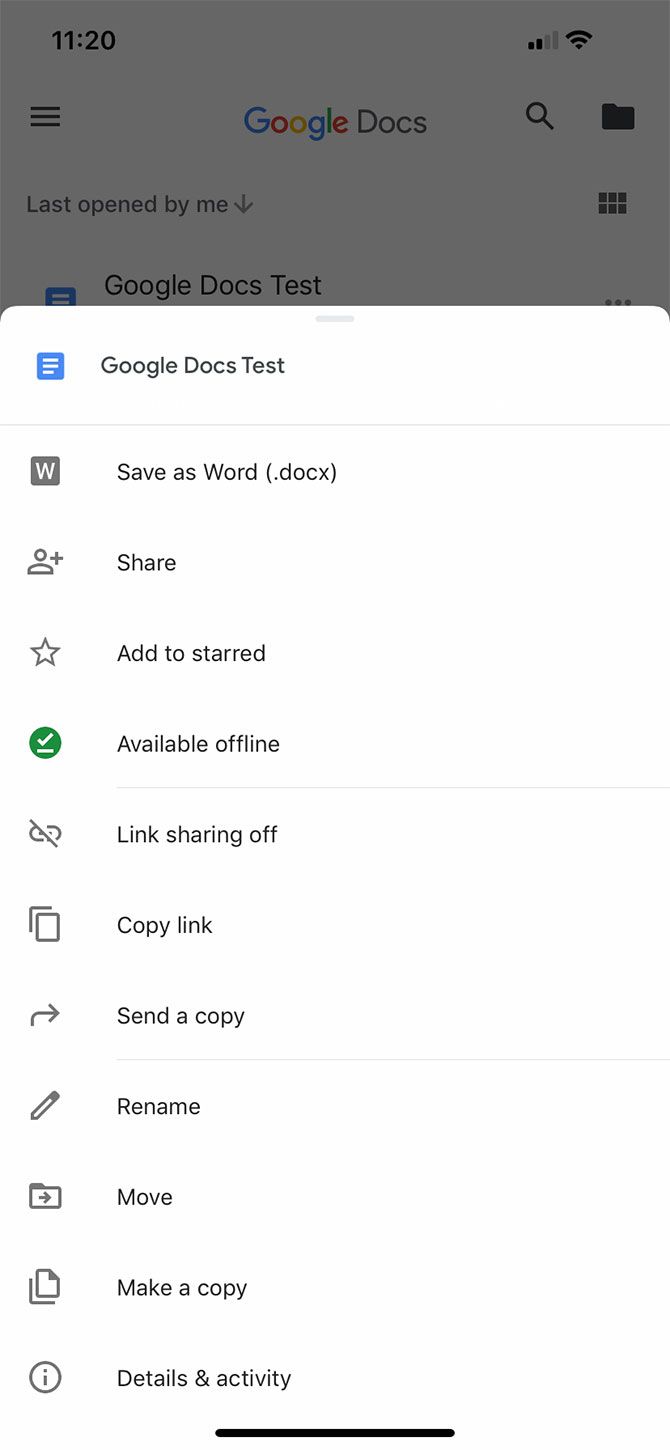The image displays a Google Docs settings page. At the top, against a grayed-out background, the time is shown as 11:20. The upper right of the screen features a data and Wi-Fi indicator, alongside an icon of three horizontal black lines representing the menu for additional options.

The main heading reads "Google Docs," accompanied by a search bar and a folder icon. Below this is the text "Last opened by me," followed by a document labeled "Google Docs test." 

A white pop-up window is prominently featured in the center of the screen with the title "Google Docs test." Within this window, there are several selectable options, including: 
- Save as Word (.docx)
- Share
- Add to starred
- Available offline
- Link sharing off
- Copy link
- Send a copy
- Rename
- Move
- Make a copy
- Details and activity

At the bottom of the screen, there's a small black-lined border with a pull tab, which can be used to adjust the visibility of the pop-up window.